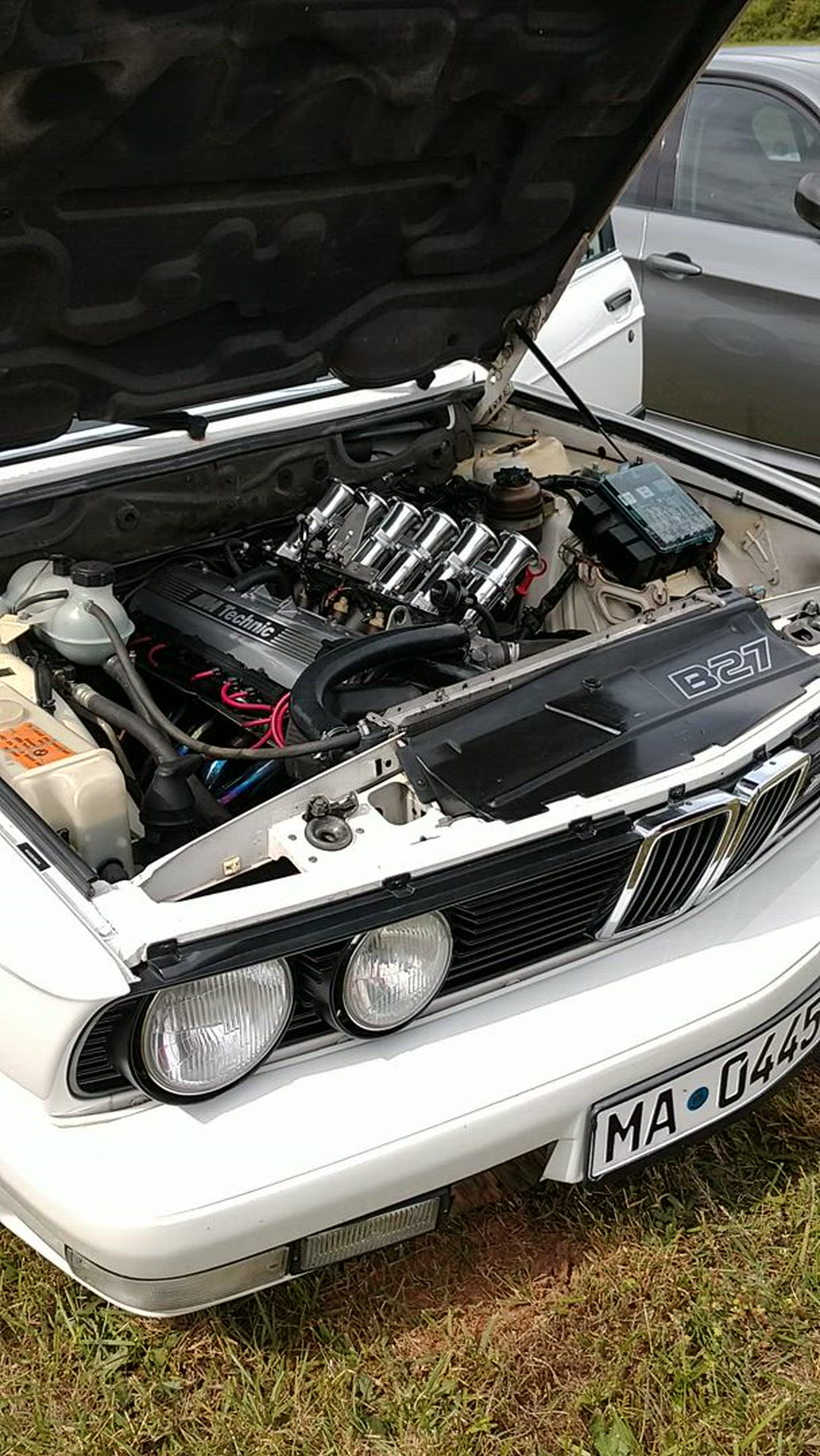The image showcases a white sports car, parked outdoors on a patch of rough, browning grass. The hood is raised, revealing a pristine, silver engine compartment lined with several components. Central to this display is the top of the engine, marked with "AW Technic" and "B27." The car's engine bay includes several distinctive features: large chrome cylinders, a fuse box with a clear plastic lid on the right, and two white liquid holding tanks on the left, possibly for windshield washer fluid and coolant. The black-lined hood is propped open by a visible supporting rod. At the front, the car boasts two round glass headlights and a black grill with vents, as well as a small, white rectangular license plate reading "MA•0445." To the right of the car, the driver's door is also wide open. Additionally, another car is visible beside it, suggesting the picture might have been taken in a car lot.